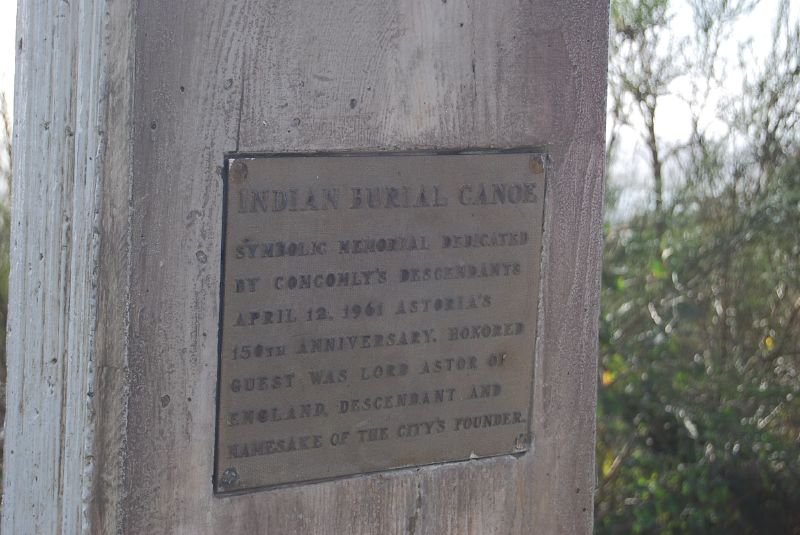The image features a close-up shot of a square, dark gray bronze plaque mounted on a lighter gray wooden board that is standing upright. The plaque bears the following inscription: "Indian Burial Canoe Symbolic Memorial dedicated by Con Comley's descendants April 12th, 1961 Astoria's 150th anniversary. Honored guest was Lord Astor of England, descendant and namesake of the city's founder." The lettering on the plaque is raised and prominent. The wood is weathered, matching the gray tones of the plaque, and is securely fastened with screws or bolts at each corner. The background reveals a wooded area with numerous trees and a gray sky, indicating a natural, serene setting. The detailed memorial commemorates a significant historical event with an emphasis on heritage and lineage.